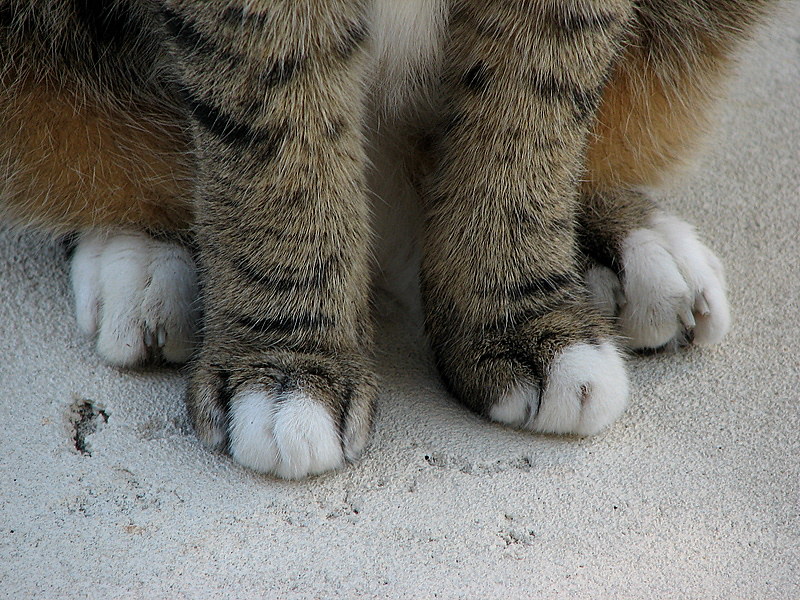This extreme close-up image captures the feet of a cat, mostly centered on its white-toed front paws. The cat is seated on a rough, mainly white surface, which appears to be either styrofoam or a concrete pad with various holes and subtle black shading, and a small brown spot in the lower left corner. The outer toes of the front paws have gray or partially gray fur with some black stripes, while the back feet, slightly tucked behind, reveal a little brown fur and a few visible claws against a background of more white. The cat's legs are a mix of tabby colors, predominantly dark beige with black streaks in random places, extending from the legs to the feet, with each toe predominantly covered in white fur. The cat sits upright, with its body partly visible, adding to the intricately patterned appearance of its fur, blending brown, gray, and hints of orange, along with the white belly fur visible between the front legs.